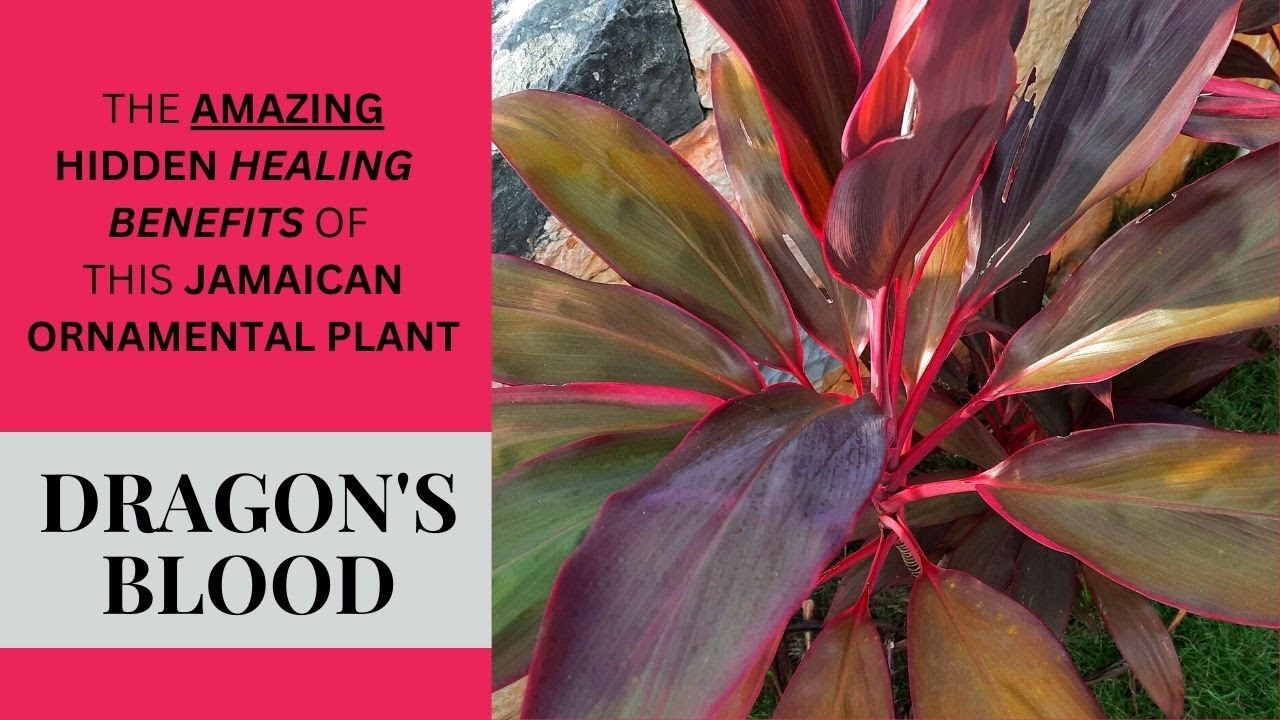The graphic features a rectangular advertisement with a bright pink background. On the left side of the graphic, text in black highlights "The amazing hidden healing benefits of this Jamaican ornamental plant." Below this text, a white stripe contains the words "Dragon's Blood." To the right of the text, a photograph showcases the plant itself, which appears edited. The plant, called Dragon's Blood, has large, firm, oval-shaped leaves. These leaves exhibit a striking mix of green and red hues, with some appearing more red throughout. The leaves have a prominent vein running through the middle and red edges, and the plant is supported by light red stems. Notably, the plant has no flowers, only its beautifully colored leaves.